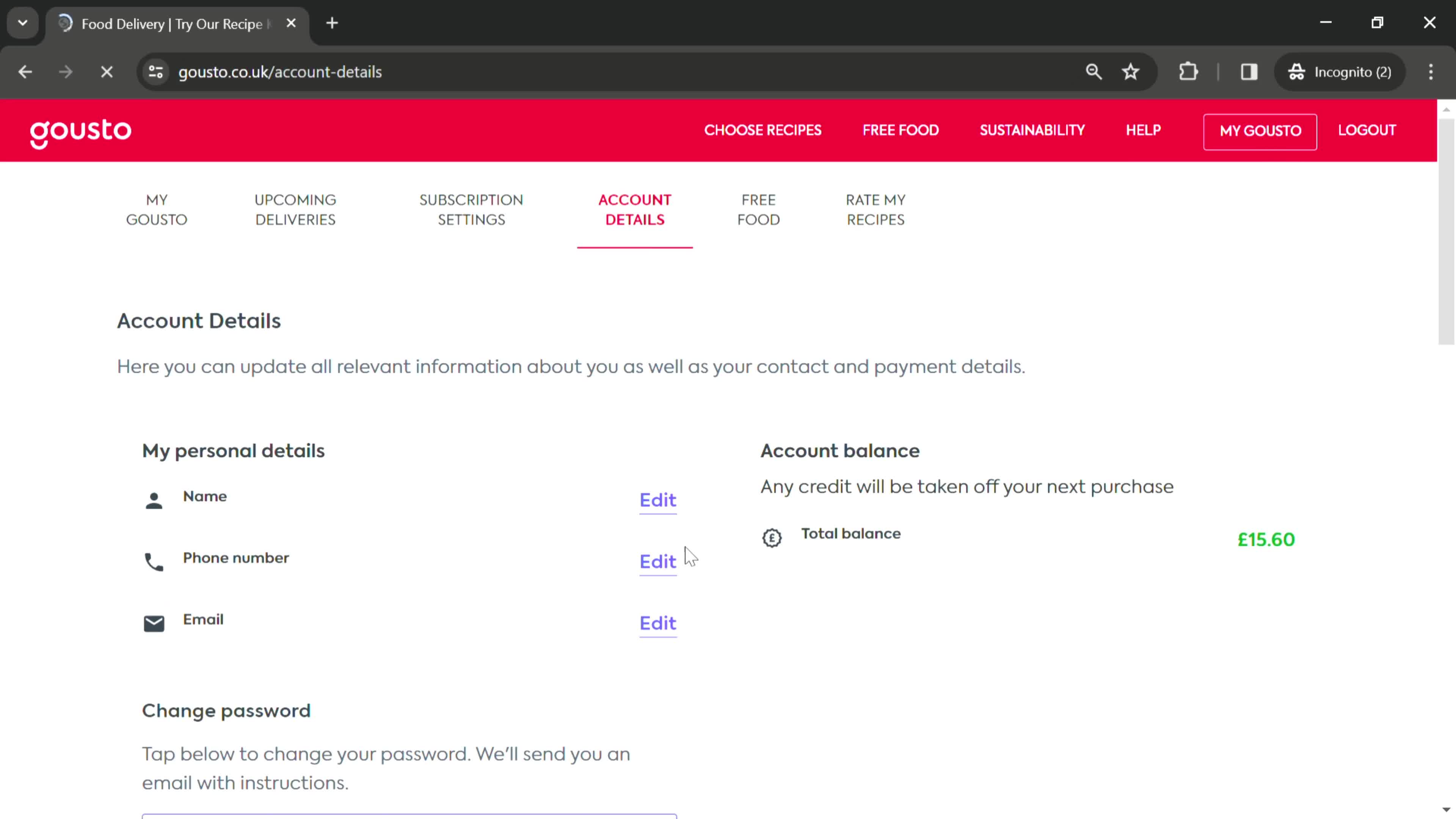The image depicts a webpage screenshot from the Gousto food delivery service, specifically centered on the "Account Details" section. In the top corner, the URL in the search bar reads "gousto.co.uk/account-details," confirming the user's location on the site. A prominent, long red rectangle occupies a significant part of the interface, which includes navigational options. 

To the left of the rectangle is the Gousto logo—a circle with a curved line beneath, resembling a stylized "G." Following the logo are menu options labeled "Choose Recipes," "Free Food," "Sustainability," "Help," "My Gousto," and "Logout." Below this navigation bar, secondary options list "My Gousto," "Upcoming Deliveries," "Subscription Settings," "Account Details" (which is highlighted in red and underlined), "Free Food," and "Rate My Recipes."

In the main section, a description reads, "Here you can update all relevant information about you as well as your contact and payment details." This text is followed by fields allowing the user to edit their personal details, including name, phone number, and email address. To the right, an account balance section details that any credit will be applied to the next purchase, displaying a total balance of £15.60 in green.